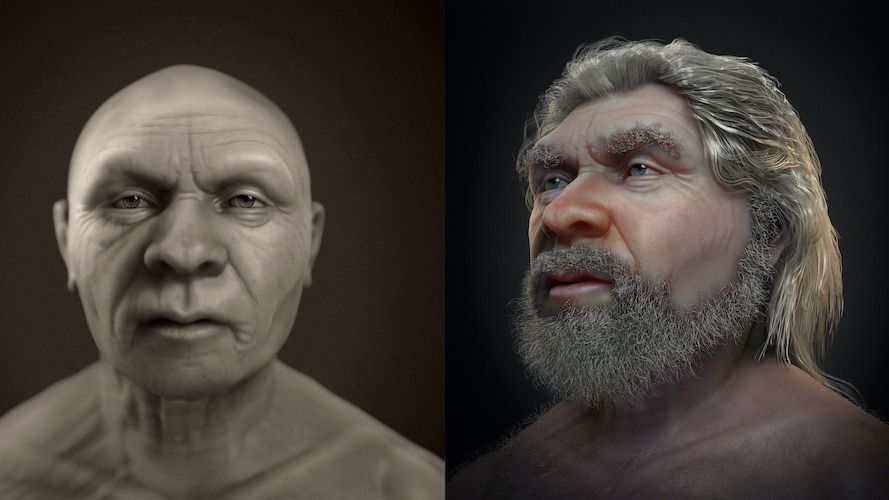The image is divided in half, showcasing a man in two different looks. On the left side, the man is bald with no facial hair, displaying a clean-shaven appearance. His eyes and nose are symmetrical, giving a distinct and recognizable visage. He has light skin, a broad nose, and full lips. Despite some shadows, he has either brown or light taupe gray eyes.

On the right side, the same man is depicted with shoulder-length hair styled in a mullet, a full beard, mustache, and bushy eyebrows, all predominantly gray with some black peppering. His blue eyes remain a focal point, accentuating his transformation. He stands slightly turned towards the left, yet his symmetrical facial features and sloping shoulders are still clearly visible. The contrast in appearance distinctly illustrates the significant changes between his bald, clean-shaven look and his more rugged, hirsute one.